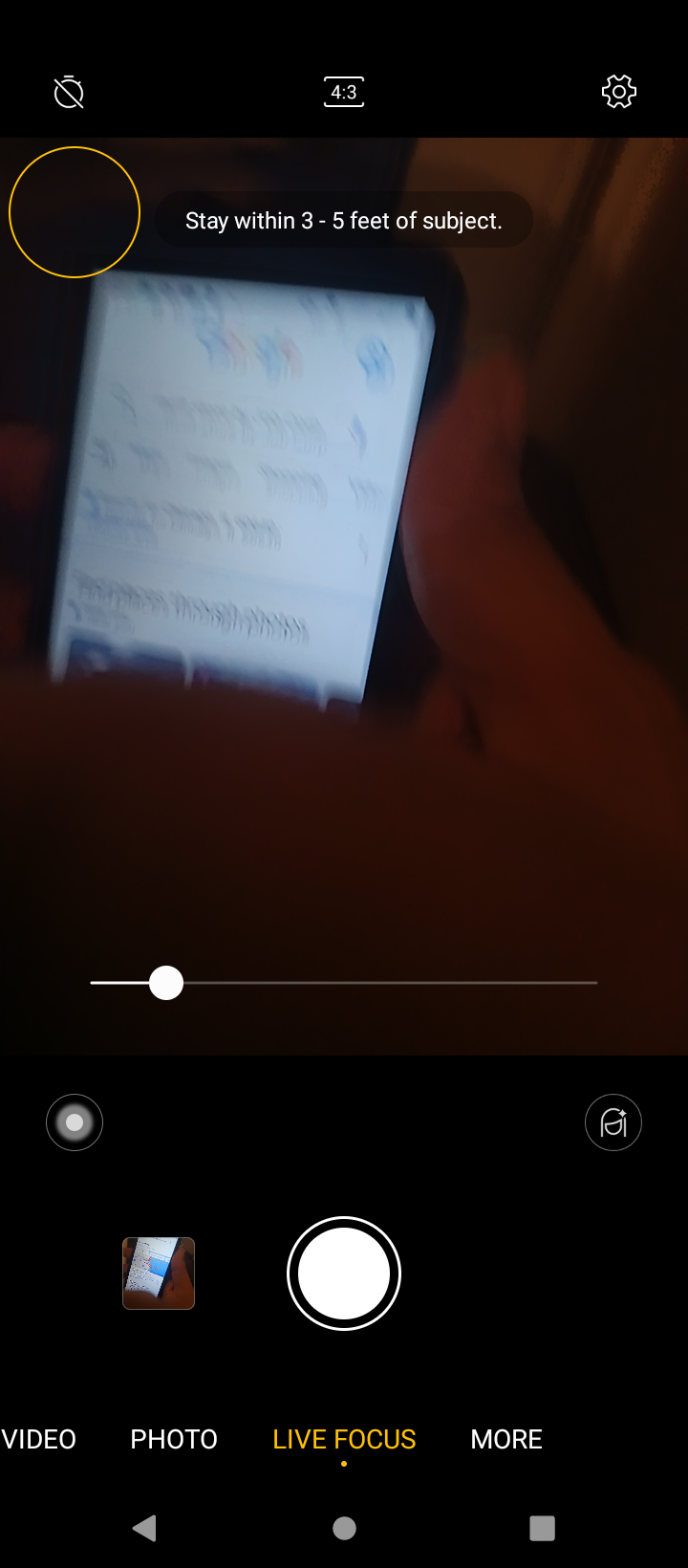This is a detailed screenshot taken from the camera app on a cell phone. At the top of the screen, three icons are visible: the left icon resembles a circle with a line through it, the middle icon displays the aspect ratio of the image being captured, and the right icon is a gear symbol indicating the settings menu. The image being photographed appears to feature a cell phone placed against a dark brown background, which could be a type of surface or setting with a rich, earthy tone. Upon closer inspection, there is a thumb visible on the right-hand side of the image being captured, suggesting that a person is holding the cell phone for a close-up shot.